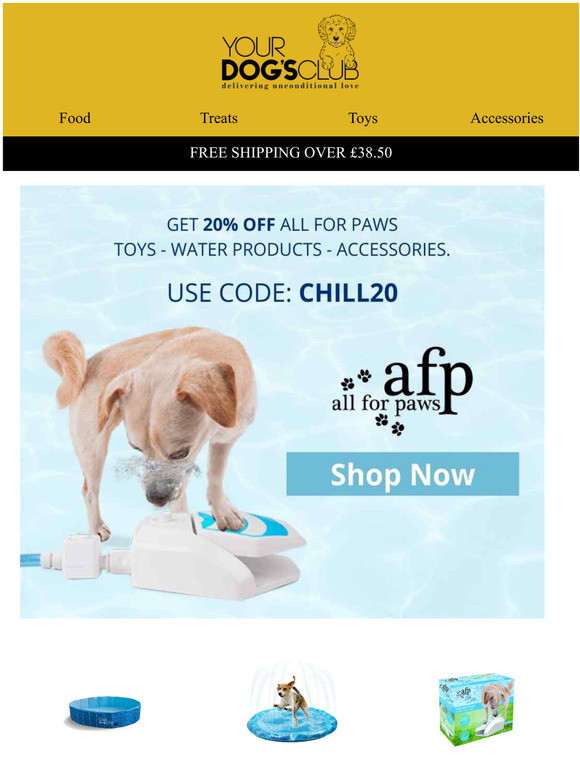This screenshot from the website "Your Dog's Club" features a detailed layout of the homepage. At the top, a dark yellow banner hosts the text "Your Dog's Club" centered, accompanied by a charming illustration of a dog playfully hanging its paws over the letters 'U' and 'B' in "Club." Directly underneath, the tagline "Delivering Unconditional Love" is prominently displayed. The navigation menu, featuring options such as Food, Treats, Toys, and Accessories, sits just below.

A black banner announces a special shipping offer: "Free Shipping over £38.50." Dominating the center of the image, the main visual showcases a small, fawn-colored dog drinking from a white water fountain apparatus connected to a garden hose. The dog activates the water flow by pressing down on a blue and white pedal with its front left paw, causing water to squirt up for the dog to drink.

A promotional message spans the image: "Get 20% Off All 4 Paws Toys, Water Products, Accessories. Use code CHILL20." Beneath this, the branding "AFP All 4 Paws" is highlighted with two paw print icons to the left of the 'A', and two more paw prints below.

Centrally located, a dark blue banner with the text "Shop Now" in bold white letters rounds out the promotional offer. At the very bottom of the image, a smaller section depicts three items: a blue kiddie pool, a blue mat that sprays water as a beagle runs through, and a box displaying the white drinking apparatus featured in the main image.